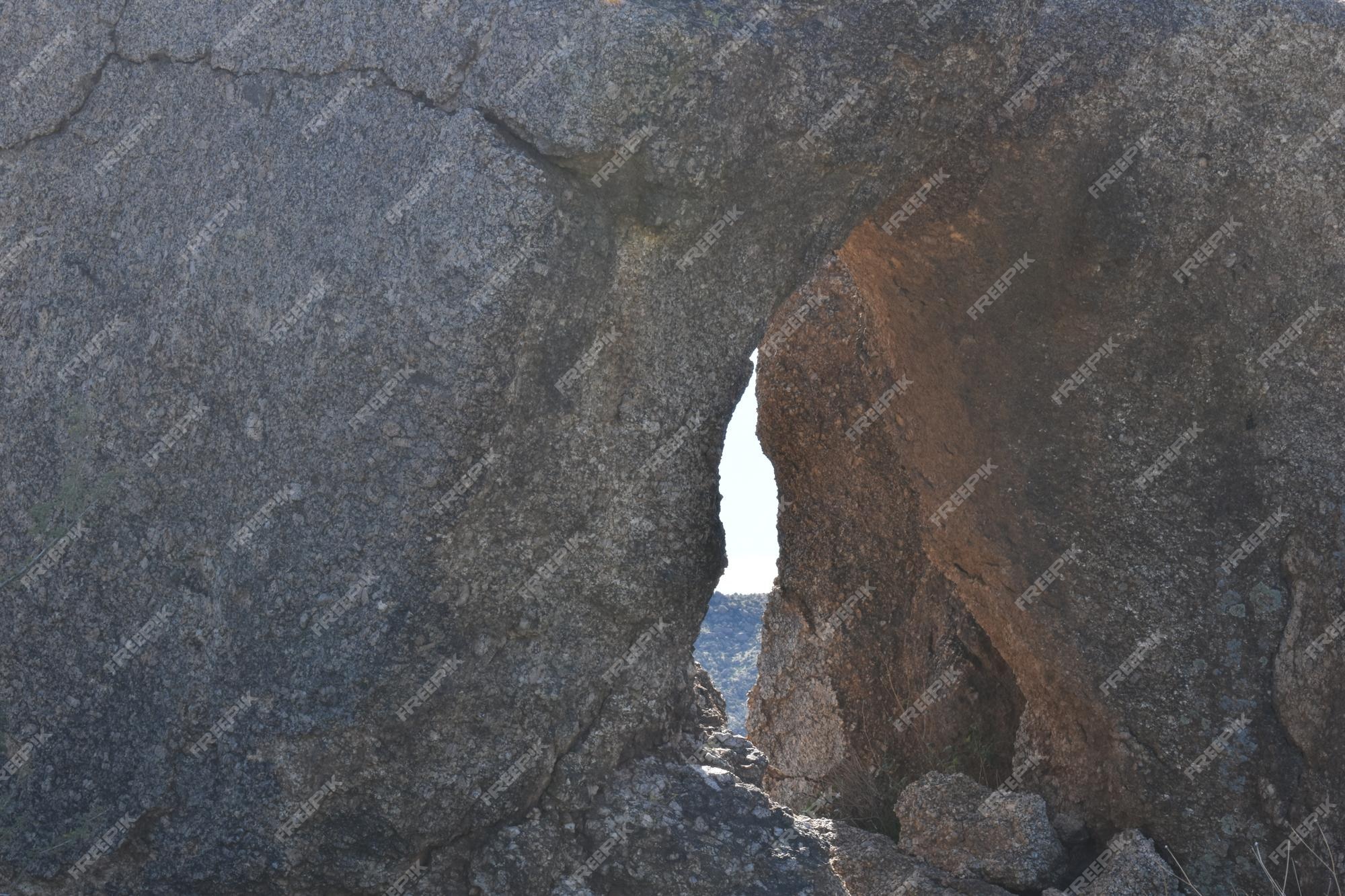The image showcases a striking outdoor rock formation characterized by a predominantly gray, textured surface interspersed with intricate lines and cracks. Centrally located is a keyhole-shaped archway or cave-like divot, creating the appearance of a miniature mountain. This archway, which has a cylindrical, triangular contour and is pointy at the top with curved sides, reveals a passage to the background. Inside the archway, the rock transitions to a brown, rust-like hue. Through the archway, a sliver of bright white sky is visible, indicating a clear, possibly cloudy day. Below the sky, the distant background features green foliage and blue waters, perhaps an ocean. The entire image is diagonally overlaid with a faint watermark that reads "FREEPIK" in rows from the left to the right, subtly marking the otherwise natural and rugged scene.